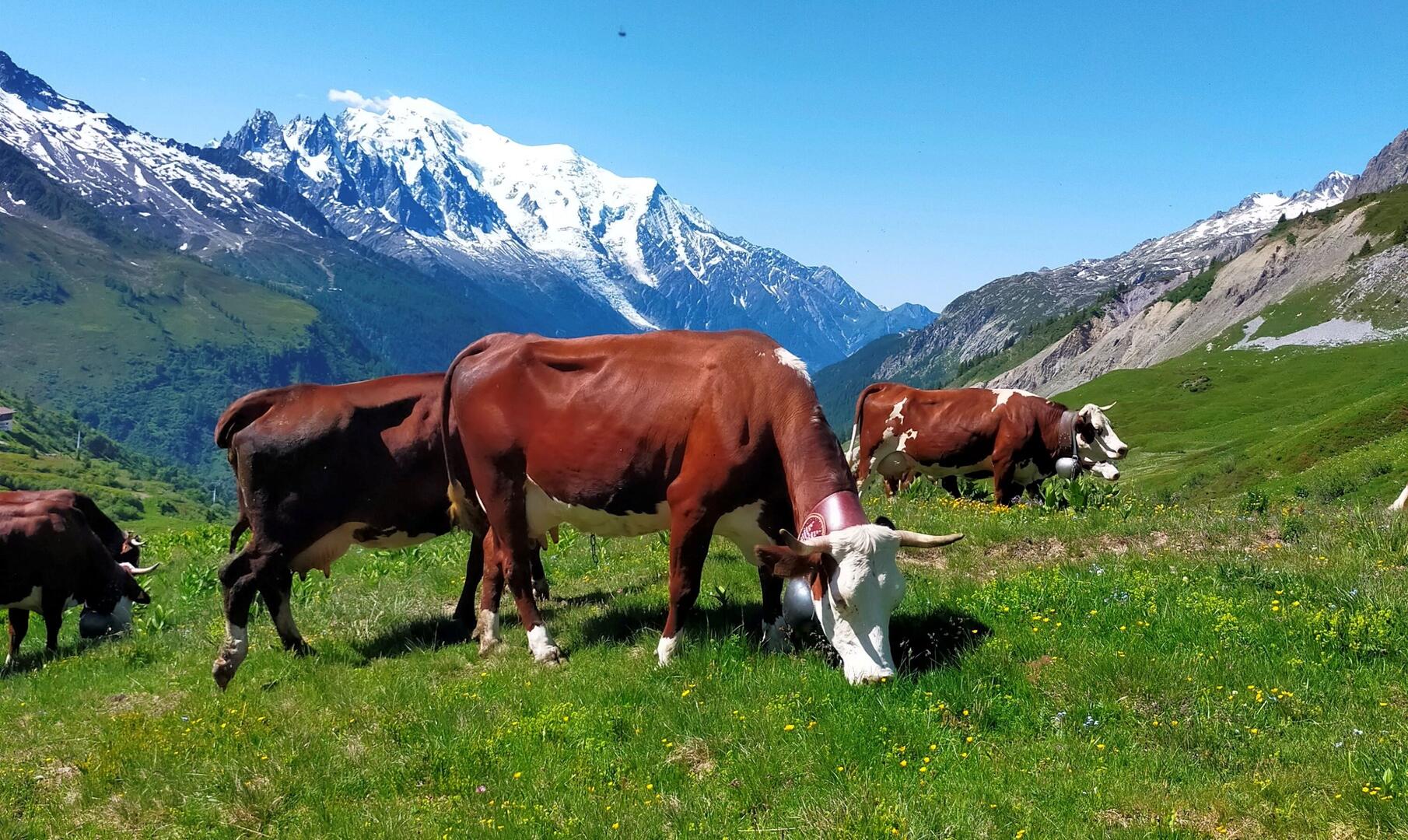In this vibrant photograph, five reddish-brown cows with white heads and horns graze contentedly in a lush, green field dotted with small yellow flowers. The gracefully undulating landscape is set against the majestic backdrop of snow-capped mountains, with larger peaks rising to the left and rocky, smaller hills on the right. The sky above is a brilliant, cloudless blue, transitioning to a lighter hue near the horizon. The foreground cow, positioned centrally, is engrossed in munching the green and lush grass, adding a lively touch to this serene pastoral scene. The cows' white markings and horns stand out crisply, contributing to the overall picturesque allure of the setting.